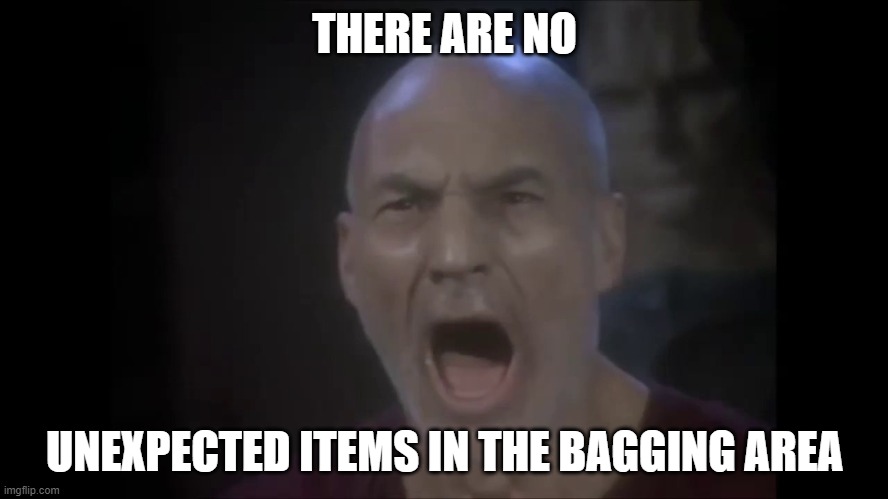This intense image from the show "Star Trek: The Next Generation" captures Patrick Stewart in his iconic role as Jean-Luc Picard. Picard is depicted in a moment of raw emotion, looking straight ahead with his mouth wide open, seemingly yelling in pain or anger. His eyes reflect the depth of his suffering. The image has black bars along the left and right sides, giving it a dramatic frame. The background is shrouded in dark shades of black and gray, adding to the stark atmosphere. Behind Picard stands a fuzzy figure, identifiable as a Cardassian—a species known for their gray skin, distinctive facial ridges, flared nose, black hair, and peculiar neck flaps. The Cardassian's ominous presence hints at the context of the scene, in which Picard endures brutal torture. The caption is overlaid with the text "There are no unexpected items in the bagging area" at both the top and bottom, a modern sarcastic twist referencing the famous scene where Picard defiantly yells, "There are FOUR lights!" resisting his torturers' attempts to make him say there are five lights when there are actually only four. This caption poignantly alludes to Picard's unyielding resistance and the psychological torment he endures.